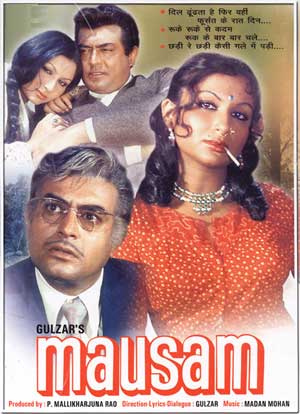This detailed movie poster, possibly from India, prominently features the title "Gozars Musam" in bold 3D red and white letters at the bottom. At the top of the poster, it credits the producers P. Malik and Harjuna Rayo, with the direction and lyrics by Gozars, and music by Madam Mohan. Dominating the center of the poster is an image of a woman on the right, wearing a red polka-dotted dress with white spots, and two thick necklaces resembling handcuffs. She tilts her head slightly to the right while holding a cigarette in her mouth. Next to her, on the left, stands a man with gray hair, glasses, and a small pencil mustache, dressed in a gray suit and looking upward to his right in apparent shock. In the top left corner, another couple is displayed; the woman leans on the man's shoulder with a seemingly drugged expression. He is also looking right and wears a suit. This ensemble suggests the movie revolves around these two couples. The woman in the center, notable for a cultural bindi on her forehead, underscores the movie's Indian heritage.